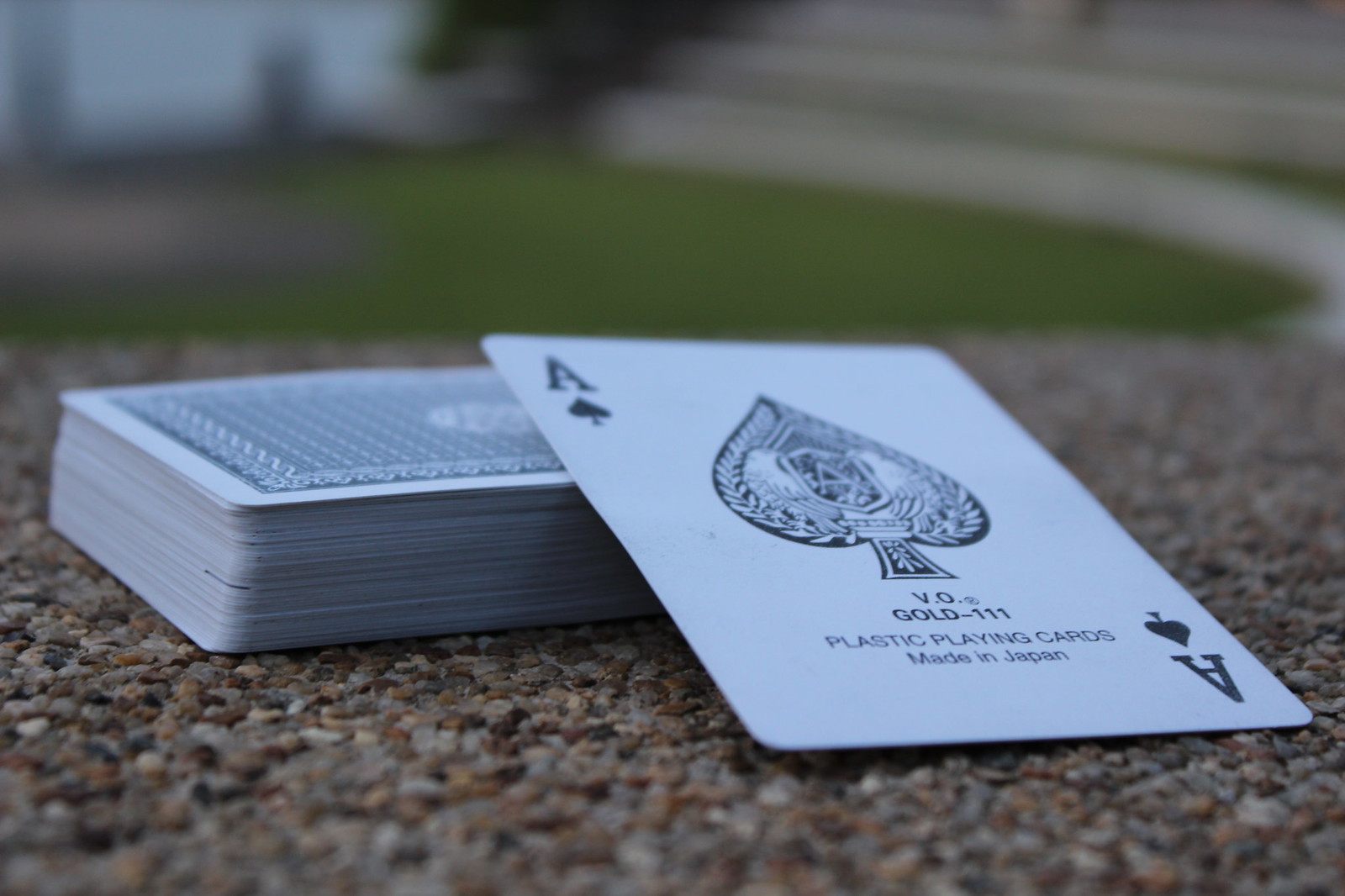In this photograph, a neatly stacked deck of cards is prominently displayed on what appears to be a coarse concrete surface, possibly a table or bench. The concrete is embedded with small rocks and pebbles in various shades of gray, black, tan, and brown, creating a textured backdrop. The background of the image is softly blurred, revealing hints of green that suggest it might be grass.

The deck of cards appears new—its edges are sharp, surfaces glossy, and overall sheen pristine. The cards are stacked face down, showcasing a blue patterned back. However, one card lies face up on top of the deck: the Ace of Spades. This card's design features a large, bold spade symbol in the center. Below the spade, text reads "VO Gold - 111, plastic playing cards made in Japan," all set on a clean white background. This intricate detail emphasizes the Ace of Spades' unique and high-quality design.